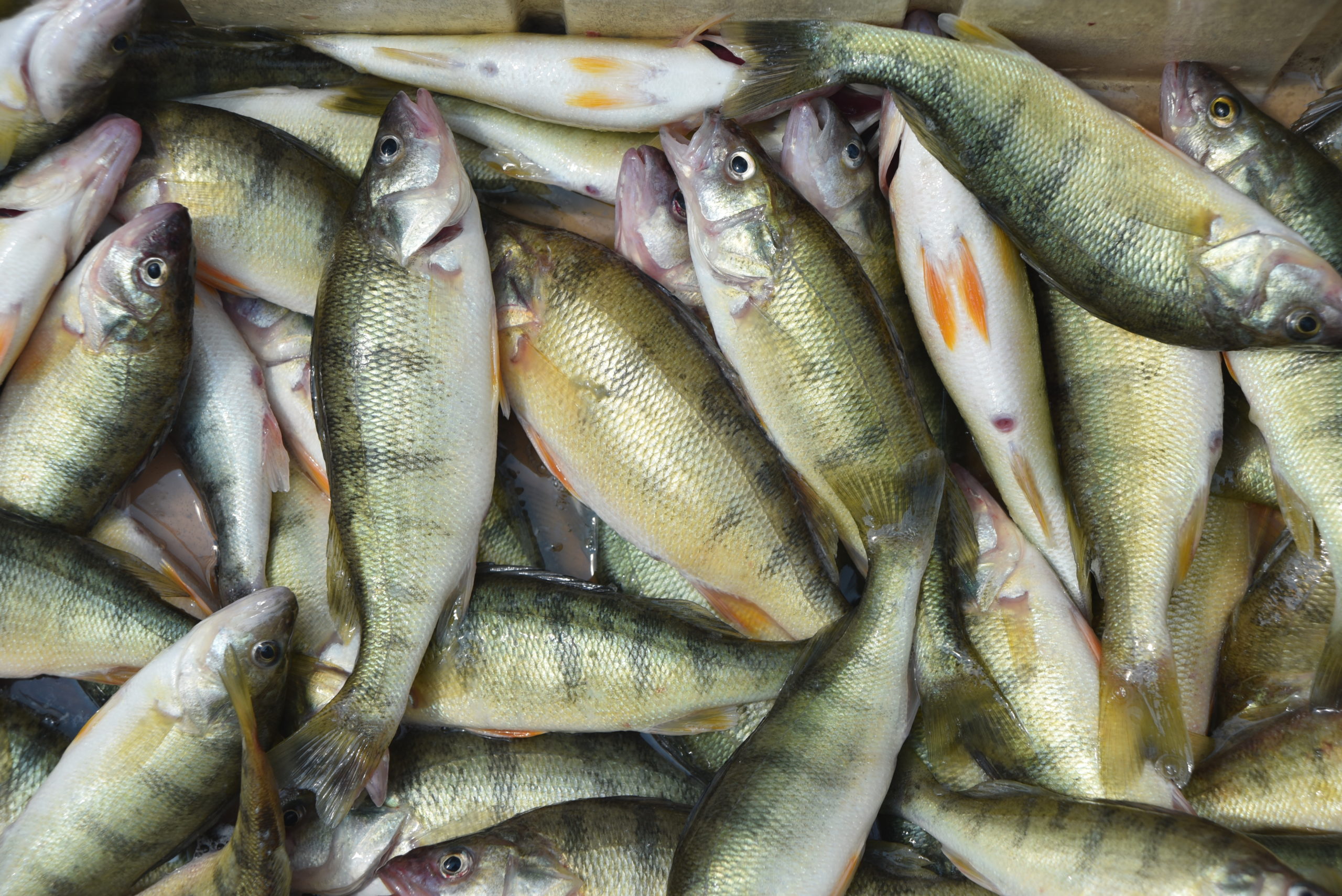The image depicts a pile of approximately 50 dead fish, stacked atop one another, likely caught by a fisherman and placed in a wooden crate or cooler. The fish exhibit a muted, army green color with a lot of scales that reflect light, giving them a slightly golden appearance. Their stomachs are predominantly white with some hints of orange, and their fins are yellow to algae-green. Each fish has silver eyes with black pupils and pink to pinkish purple mouths, some open and some closed. A light source illuminates the scene, accentuating the fish's scales and giving the realistic image a somewhat reflective quality. One noticeable fish on the left stands out, oriented vertically, and appears to be about one foot long.